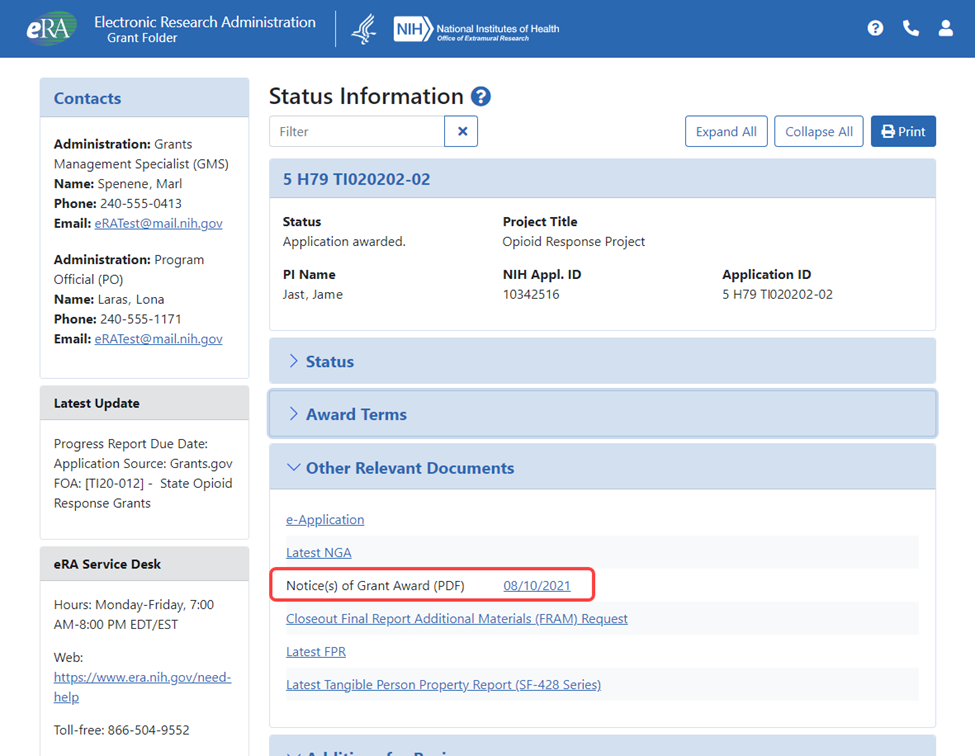The image features a dark blue border at the top, adorned with a logo consisting of a lowercase 'e' and an uppercase 'RA' on a green background. The upper left corner displays the text "Electronic Research Administration Grant Folder" with the abbreviation "NHI" representing the National Institutes of Health. Adjacent to this text are three icons: a circle with a question mark, a phone, and a person.

On the left side of the blue box, the word "Contacts" is prominently displayed. Below this title, the contact details for two administrators are listed. 

First is the "Grants Management Specialist (GMS)", named Merle Spanier. The contact information for Merle Spanier includes a phone number, 240-555-0413, and an email address (not specified in the provided text). 

Next is the "Program Official (PC)", named Loner Loris. The contact information listed for Loner Loris includes a phone number, 240-555-1171, and an email address (also not specified). 

Beneath these contacts, the text "Latest Update" is mentioned, indicating recent changes or information.